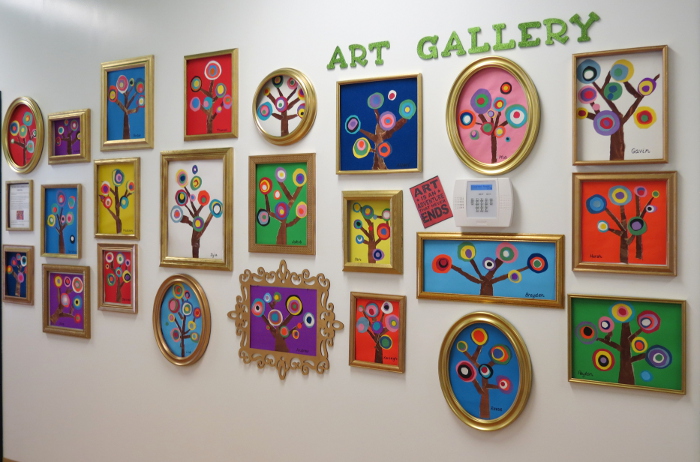The image depicts a children's art gallery showcased on a white-gray wall. At the top, "ART GALLERY" is prominently written in green capital letters. Below, various gold frames encase the artwork, with shapes including ovals, circles, squares, and rectangles both in landscape and portrait orientations. One particularly ornate rectangular frame stands out with its antique-like carvings. Each framed piece features a tree with a brown trunk and branching limbs, adorned with vibrant orbs in a rainbow spectrum of colors—greens, purples, reds, oranges, whites, yellows, and multiple shades of blue and green. The backgrounds of these pieces are equally colorful, ranging from torch red to dark blue, purple, yellow, green, white, and pink. All the artworks appear to be created in a similar, meticulous style, possibly by the same person, giving the gallery a cohesive and lively appearance. Light casts shadows on the wall, adding depth to the display. Additionally, each piece has a name written at the bottom, adding a personal touch to the collection.